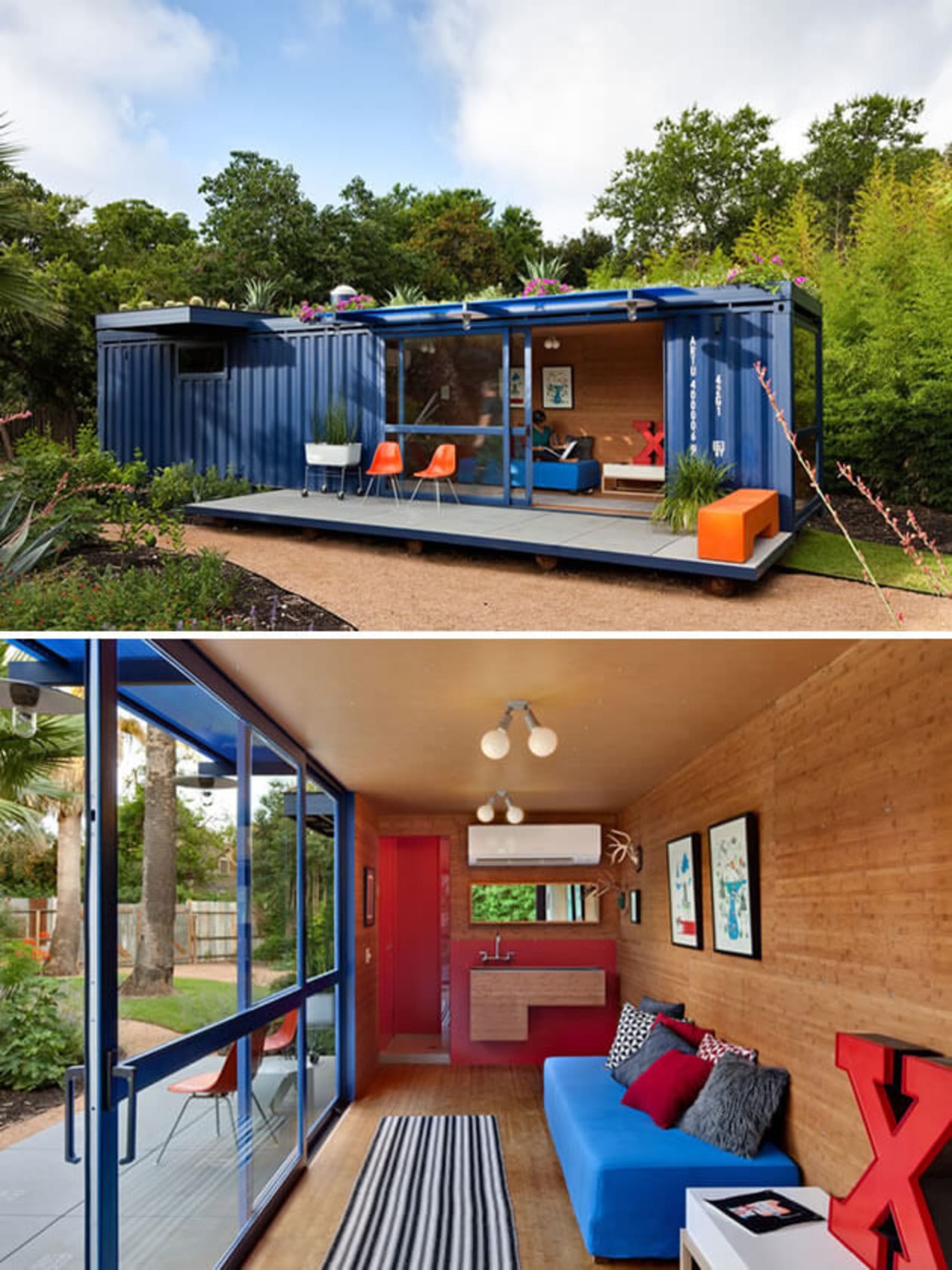The image features two color photographs of a converted blue shipping container used as a small living space or den. The top photograph showcases the exterior, with the container set amidst a garden or yard, complete with a small patio and sliding glass doors that open onto a porch. Two orange chairs sit on the patio, flanked by planters with green plants, and there are additional plants atop the container. The surroundings include trees and other garden elements, suggesting a secluded and tranquil environment. The scene appears to be taken during the middle of the evening, as indicated by the daylight and clouded sky.

The bottom photograph reveals the interior of the shipping container, highlighting a cozy living space. Inside, a blue couch with pillows rests against wooden-paneled walls and a wooden floor. There is an area rug on the floor, and a table adorned with a prominent red "X" on it. A small counter with a sink is visible, and a room beyond with a red door suggests additional space. Light fixtures hang from the ceiling, and the overall ambiance of the interior is warm and inviting.